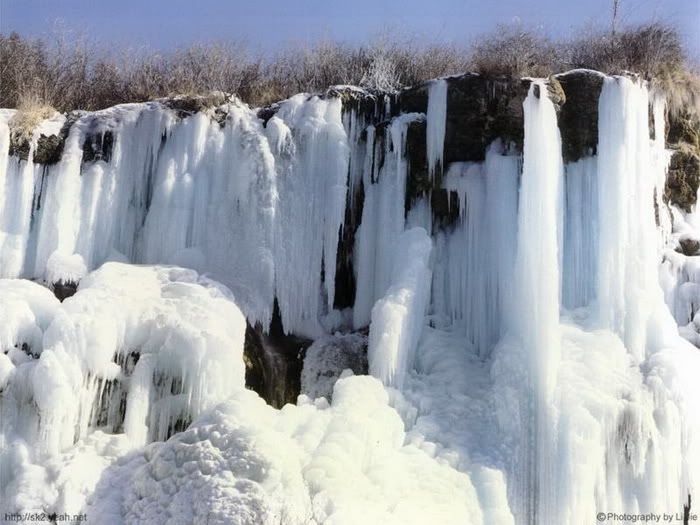The image is a large, square, stock photograph capturing a striking winter scene dominated by a frozen waterfall. Clear blue sky occupies the topmost portion of the picture, with bare trees extending below it, devoid of leaves. Beneath the trees, a massive cliff covered in dead grass and sparse vegetation forms the backdrop. Cascading down from the cliff's edge are spectacular, massive ice formations where the waterfall has entirely frozen, creating intricate icicles that stretch from the top to the bottom of the image.

Prominently centered in the photograph is a watermark with "Photobucket" emblazoned in white letters, accompanied by a white circular logo situated to the left. Directly below this watermark is an advertisement, also in a white rectangle, reading: "Protect more of your memories for less!" At the bottom of the image, more jagged, snowy rock formations can be seen, completing the frozen landscape. The photograph is finalized with a small copyright symbol noting, "Photography by Lily."